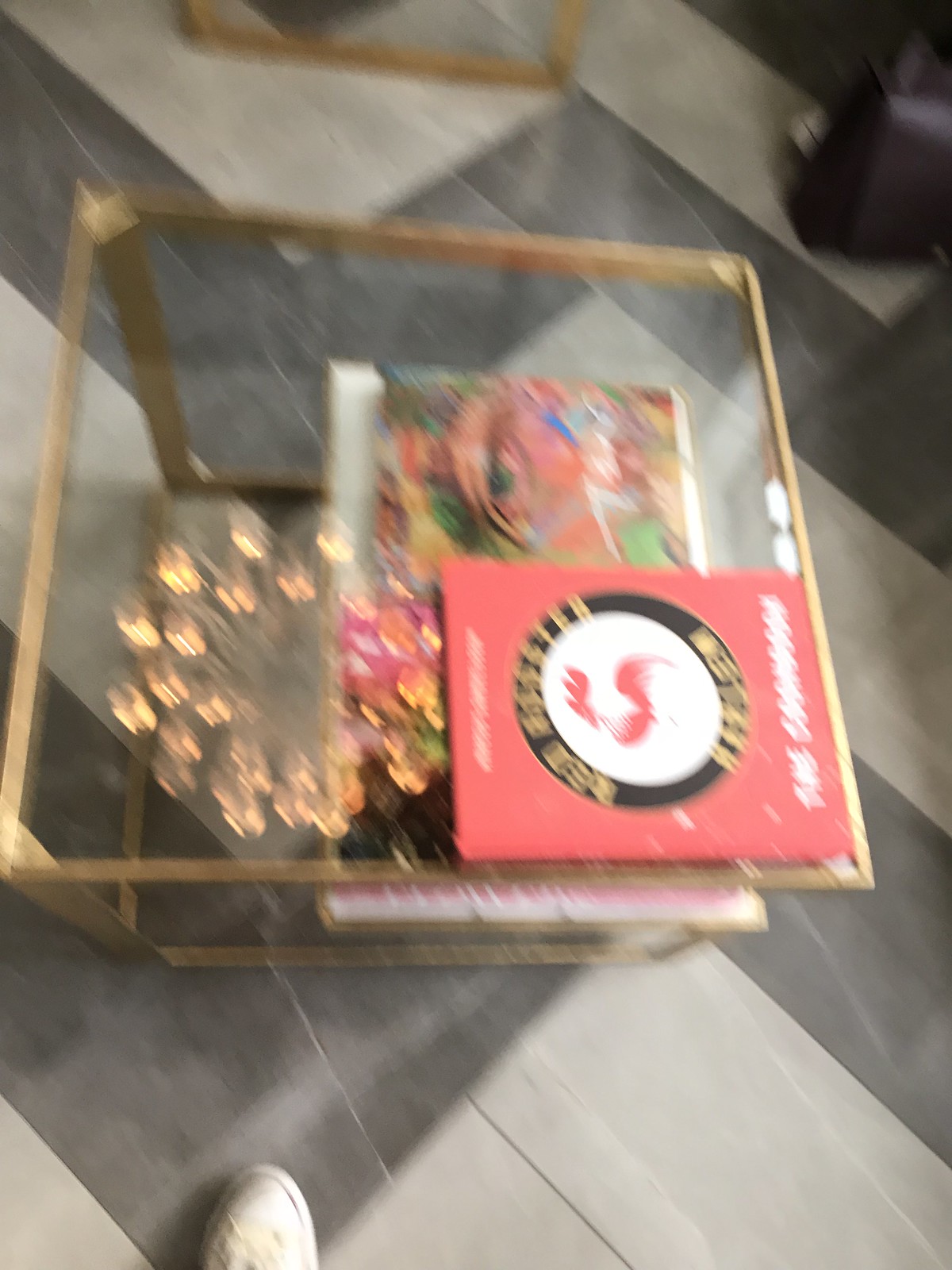The image showcases a table with a clear glass top and ornate gold-trimmed edges, although the photograph itself is quite blurry, making fine details difficult to distinguish. Atop the table sits a prominent pinkish book, its title and text rendered unreadable due to the blurriness. Surrounding the book are various other objects, each differing in color, shape, and size, but their specifics remain indistinct. In the bottom left corner of the image, the front part of a human left foot is visible, clad in a white sneaker and set against a gray floor.